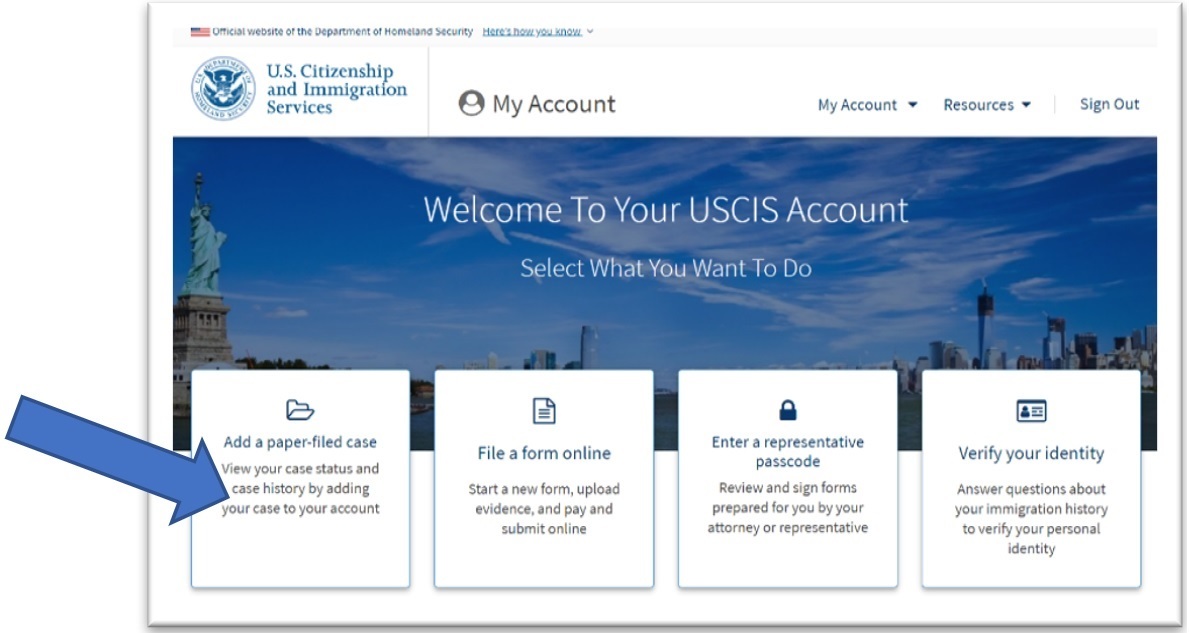Screenshot of a USCIS Account Dashboard

A screenshot of a computer interface features prominently in the image. At the very top, a white background displays the header for the official website of the Department of Homeland Security. In the upper left-hand corner, an American flag icon is accompanied by text declaring the site’s official affiliation with the Department of Homeland Security. To the right of this, blue underlined text reads "Here's how you know," with a drop-down option for further details.

Directly below this header, a seal representing the U.S. Citizenship and Immigration Services (USCIS) is visible. Adjacent to the seal, text reads "my account," followed by navigation options including a "my account" drop-down, a "resources" drop-down, and a "sign out" option further to the right.

The central portion of the screen showcases a serene image of a blue sky scattered with white clouds. On the left side of this central image, the Statue of Liberty stands majestically. On the right side, several skyscrapers rise towards the sky, creating a striking contrast against the clouds. Between these landmarks, large text in the center of the image greets the user: "Welcome to your USCIS account. Select what you want to do."

At the bottom of the screen, four square boxes present different action options for the user. The first box, highlighted with a prominent blue arrow, reads "Add a paper filed case. Enter your case status and case history by adding your case to your account." The second box invites users to "File a form online." The third box provides the option to "Enter a representative passcode." Finally, the fourth box instructs users to "Verify your identity."

This detailed layout encapsulates a user-friendly interface designed to aid individuals in managing their immigration and citizenship needs through the USCIS online account system.